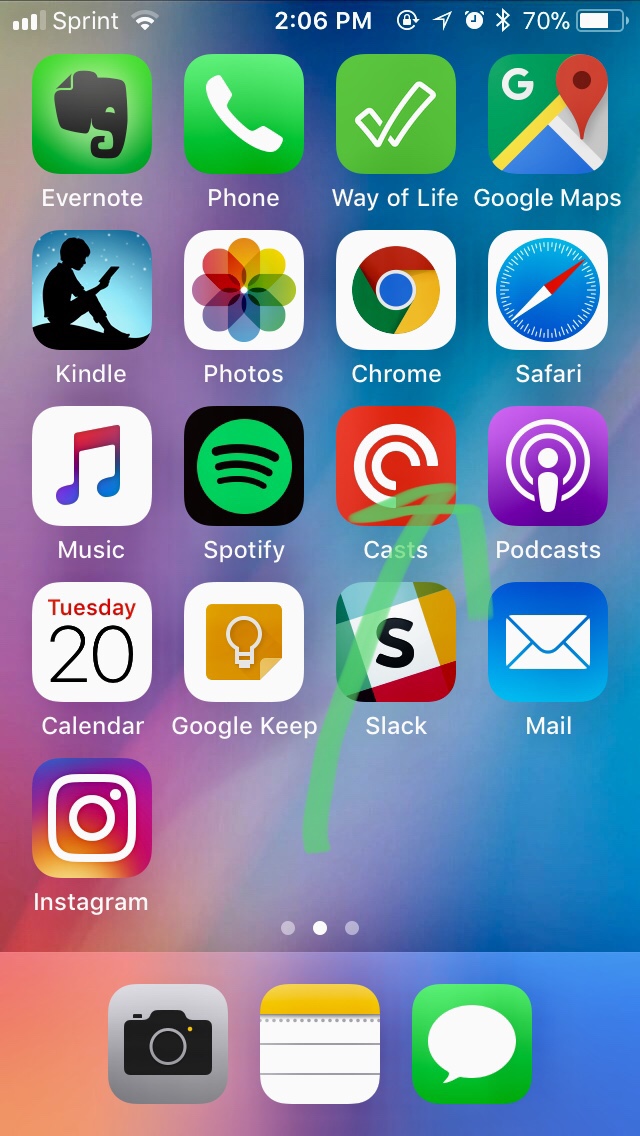This screenshot captures an iPhone home screen showcasing an array of popular applications. The backdrop features a generic, colorful gradient of blue, purple, and orange hues, with no distinct image, adding a vibrant yet subtle ambiance to the display. 

Starting from the top left and moving to the right, the visible apps are:
1. **Evernote** - Nestled in the upper left corner, known for its green elephant logo.
2. **Phone** - The classic green telephone receiver icon.
3. **Way of Life** - An app often used for habit tracking.
4. **Google Maps** - The staple navigation app.
5. **Kindle** - Amazon's ebook reader app, identified by its black silhouette of a person reading under a tree.
6. **Photos** - Featuring a multicolored flower icon.
7. **Chrome** - Google's web browser, symbolized by a colorful circle.
8. **Safari** - Apple's own web browser, depicted by a blue compass.
9. **Music** - Represented by a music note.
10. **Spotify** - The green circle with black sound waves logo.
11. **Casts** - The app highlighted by a green arrow, indicating its importance.

Continuing downward, the apps listed are:
1. **Podcasts** - Represented by a purple icon with a white microphone.
2. **Calendar** - Displaying the date in red and white.
3. **Google Keep** - A yellow icon resembling a sticky note.
4. **Slack** - The collaboration tool marked by a colorful hashtag.
5. **Mail** - The ubiquitous blue envelope.
6. **Instagram** - Identified by its gradient camera icon.

At the bottom dock, the staples include:
1. **Camera** - Recognized by a camera lens icon.
2. **Notes** - The yellow and white notepad icon.
3. **Messages (iMessage)** - The green speech bubble icon, typical for text messaging.

Indicators at the top of the screen show:
- The carrier, **Sprint**, with two bars of service.
- A **Wi-Fi** signal.
- The current time **2:06 PM**.
- Icons for **Lock**, **Location**, **Alarm**, and **Bluetooth**.
- The battery at **70%**.

Towards the bottom, the ellipsis signifies the existence of two additional home screens filled with more apps. The overall layout is a typical iPhone setup, brimming with widely used applications, each contributing a splash of color to the home screen.